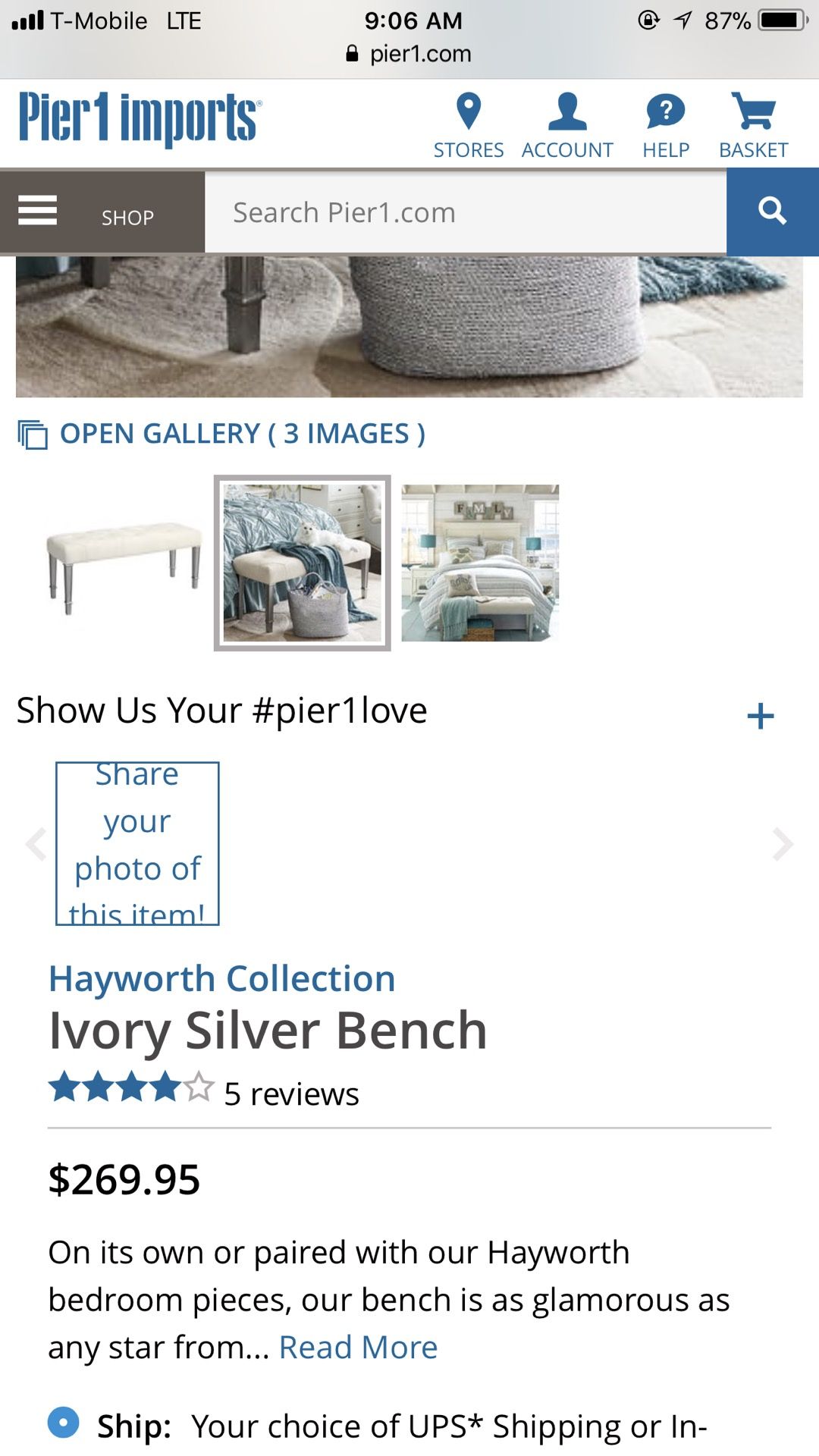Here is the revised descriptive caption for the image:

---

A screenshot from a mobile device displays a page from the Pier One website. At the top of the screen, there's a light gray status bar indicating cell reception, showing "T-Mobile" and "LTE" in capital letters. The time is displayed as 9:06 AM at the center, with a padlock icon beside the website's URL "Pier1.com." On the right side, the battery status reads 87%.

Below this, the main webpage features a white background with "Pier 1 Imports" highlighted in blue text. Navigation options are visible, including "Stores," "Account," "Help," and "Basket." The page contains a search bar within a gray background labeled "Shop" in white text, followed by a functional search bar with the prompt "search Pier1.com" and a blue square with a white magnifying glass icon at the end.

Further down, the text "Open Gallery (3 Images)" is displayed, indicating the presence of three images beneath it. These images showcase a bench styled in various bedroom settings, enhancing the visual appeal of the furniture.

Under the images, there is a promotional text "Show us your Pier" followed by the hashtag "#Pier1Love," encouraging customers to share photos of the item. The product description reads "Hayworth Collection Ivory Silver Bench" along with a rating of four out of five stars based on five reviews. The price of the bench is listed as $269.95.